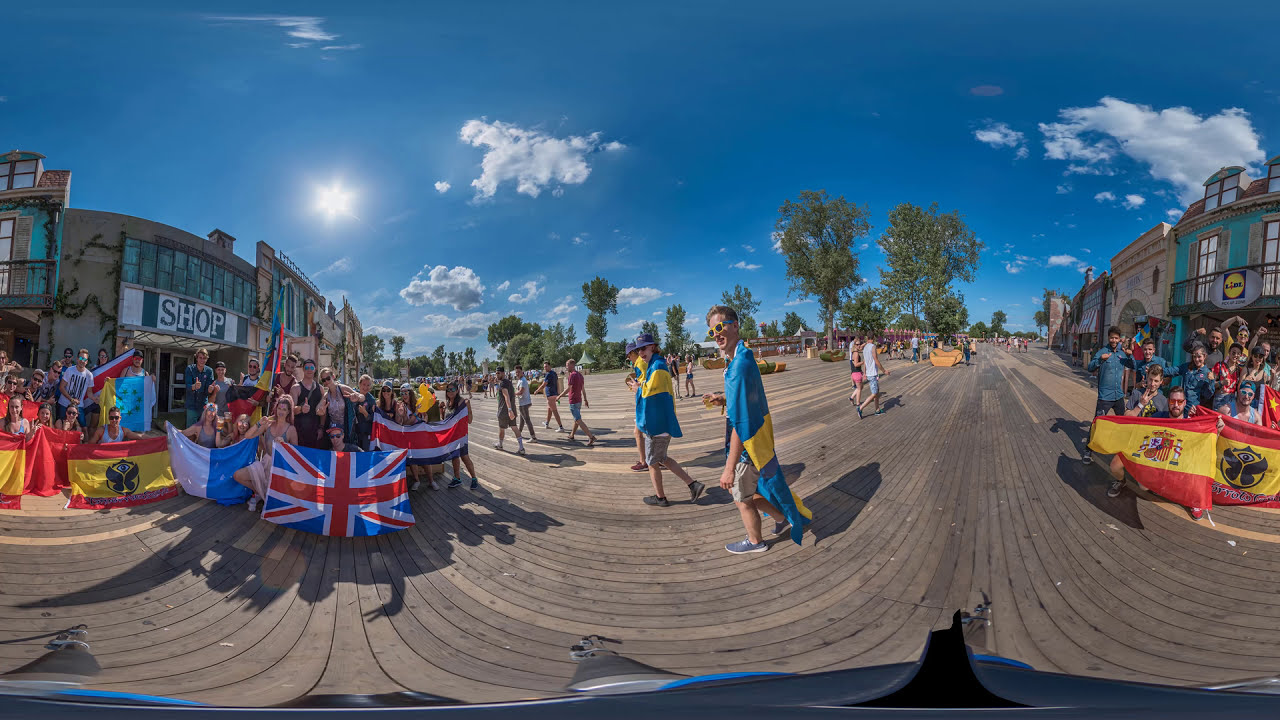The image captures a vibrant market town scene in the UK, characterized by a notable level of distortion, suggesting it was taken with a 360-degree or ultrawide lens. This creates a surreal and warped appearance, especially evident in the wooden walkway that seems to bend dramatically towards the horizon. The right-hand side features a series of shops, while the left side shows a bustling crowd of people holding various flags, including the British flag and possibly the Ukrainian flag, along with red and yellow flags. A man in a blue parka stands prominently in the middle of the image amidst this busy scene. The sky above is a brilliant blue, dotted with puffy white cirrus and nimbus clouds, and a sun flare brightens the upper left quadrant. In the distance, beyond the crowd, more shops and green trees are visible, enhancing the feeling of a bright, clear day filled with activity and national pride.